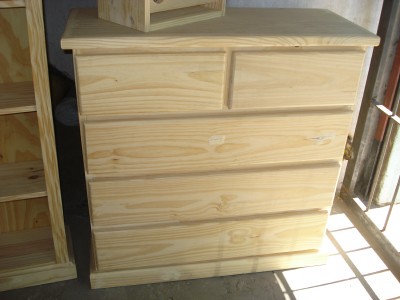The image is an indoor color photograph depicting an unfinished dresser composed of natural wood, possibly maple or pine. The dresser features three long, rectangular drawers from the bottom to the middle and two smaller drawers just below the top. All five drawers are pull-out style but lack handles or pulls. The wood is in its raw, unstained state with no primer or wood coat applied, revealing a simplistic and unembellished design. The dresser is situated on a concrete floor, beside part of an unfinished bookcase, suggesting a workshop or construction setting. Additionally, there appears to be a box or similar object made of the same type of unfinished wood resting on top of the dresser. In the background, portions of a gate and a large window with sunlight streaming through are visible, indicating a dimly lit environment.